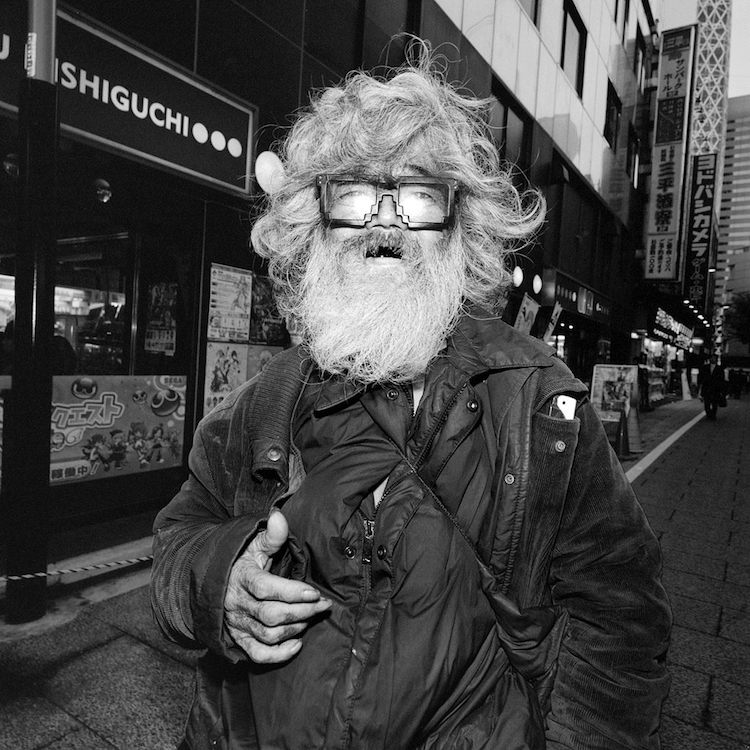This intricate black-and-white photograph captures an elderly gentleman with bushy, curly white hair, a full mustache, and a very long, bushy beard. He is wearing pixelated black glasses with thick rims, reminiscent of designs from video games like Minecraft. The man, who is standing in the middle of the image, is donning two black jackets—an outer buttoned jacket left open and an inner zipped one, possibly with various items like a pocket knife or a comb tucked into his chest pockets. He appears to be situated on a street in Japan, as evidenced by the Japanese text on shop signs and posters in the background. The shop directly behind him bears the name "SHIGUCHI," and while there is a hint of sky visible at the top right of the image, the overall setting is distinctly urban and outdoor. The man's open-mouthed expression suggests he might be speaking or in mid-thought as he gazes straight ahead.